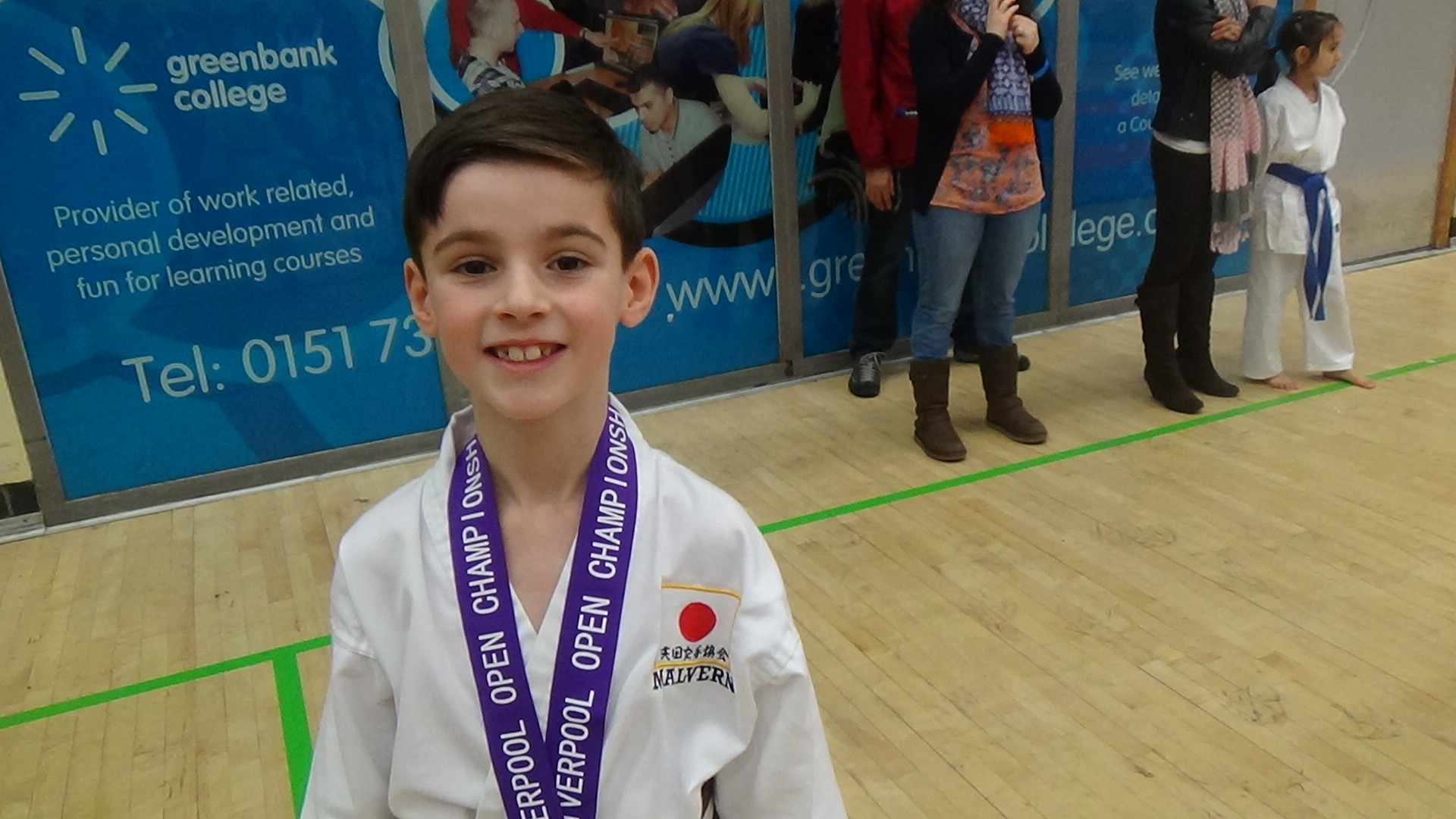The image depicts a joyful young boy standing in a gym, proudly wearing a white karate gi with a ribbon around his neck that reads "Liverpool Open Champs." His brown hair and radiant smile highlight his excitement. The gym features a light oak floor, and behind him, there are other participants, including a girl in similar attire with a blue belt, as well as some parents. Along the blue wall behind them, a sign reads "Green Bank College: Provider of Work-Related Personal Development and Fun for Learning Courses," accompanied by contact details. The scene captures the celebratory atmosphere of a martial arts event.